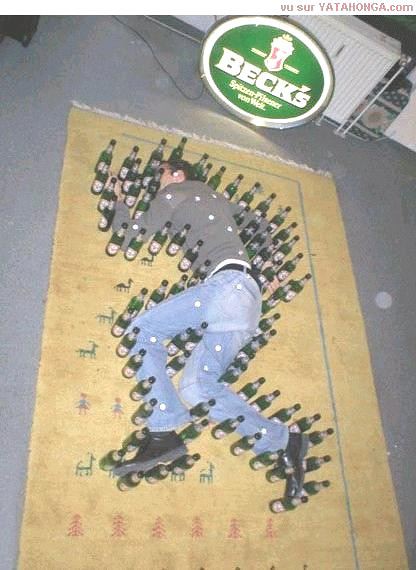The image depicts a man lying on a tan-colored rug, which features rows of small red Christmas trees, green reindeer, and light blue borders on the top and right sides. The rug is laid out on a gray concrete floor. The man, appearing to be passed out, is positioned with his head toward the top of the image and his feet toward the bottom. He lies somewhat on his stomach and side, with his left arm extended in front of his face and his right arm behind him. His left leg is straight, while his right leg is bent back. He is dressed in a gray shirt, blue jeans, and black shoes with a black belt. His entire body is outlined by an arrangement of beer bottles, resembling a chrysanthemum-scene outline, which continues around his face, arms, and between his legs. In the upper right-hand corner of the image, partially in the background, is a round green sign with white lettering that reads "Beck's," including some smaller, indecipherable text. The sign appears above a few white cabinets.